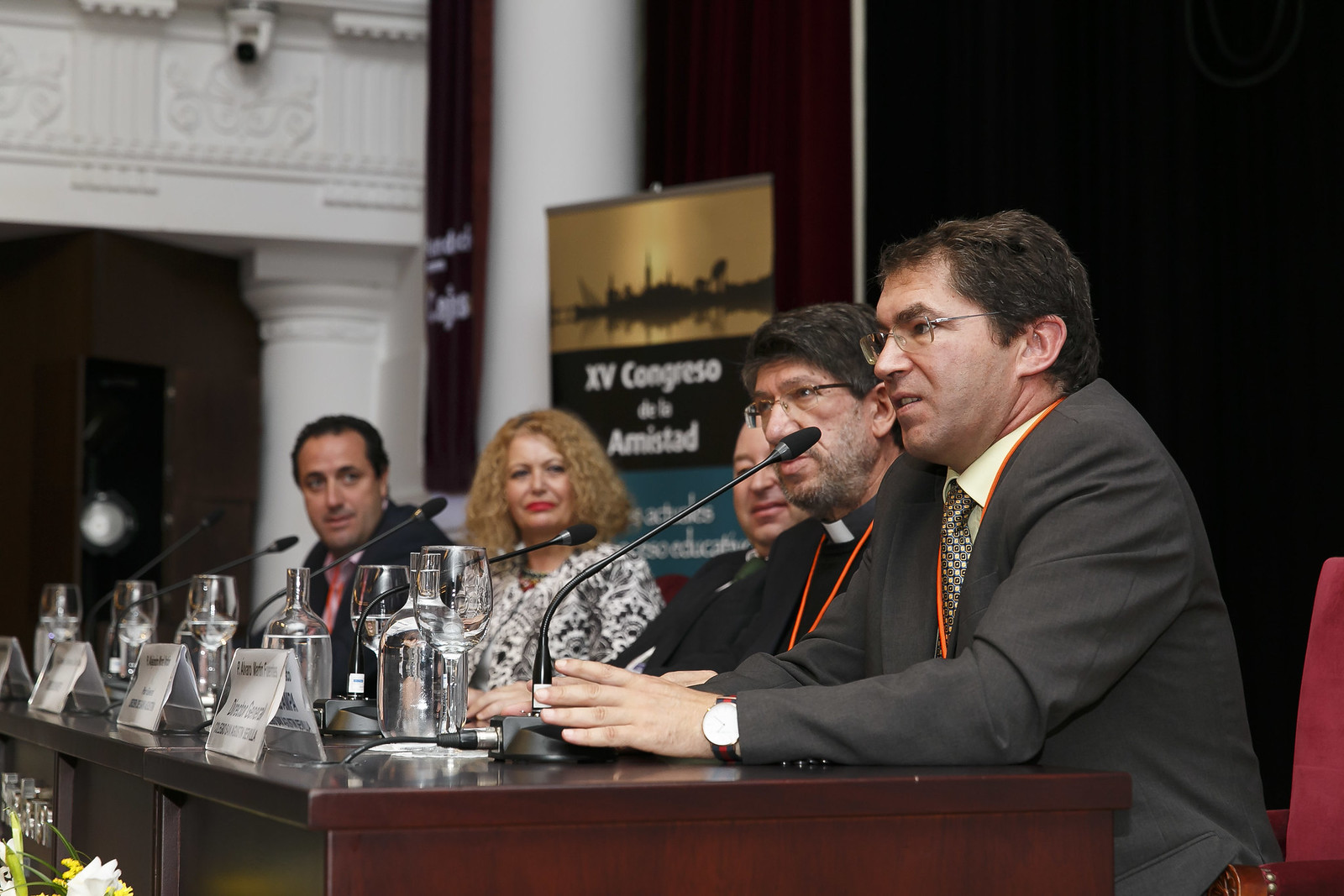A detailed caption for the described image could be:

"A group of individuals are seated at a long brown table in a large hall, captured from a left-front angle. At the forefront sits a man in a gray suit and white shirt, identified by his orange lanyard and black-framed glasses. He has both elbows resting on the table, with a thin black microphone positioned in front of him. Beside him, a man with short dark hair, also wearing glasses and a priest's collar, looks ahead. Partially visible behind them is another man, whose upper body is cut off due to the angle of the photograph. Further along the table sits a woman with light brown curly hair, adorned in a white and black dress, her face accentuated by red lipstick and makeup. She directs her gaze towards the man at the far end. Next to her, a younger man with short dark hair and a black jacket also looks towards the same direction. In front of each individual are white cards and wine glasses neatly placed on the table, indicating assigned seating arrangements or role cards for the event."